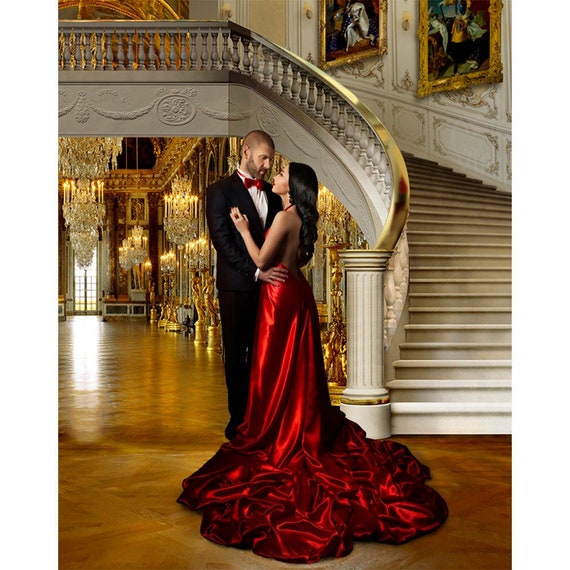In this professionally shot, full-color photograph taken indoors, a stunning Caucasian couple stands amidst a luxurious setting. The man, with a thin beard, short hair, and dressed in a sharp black tuxedo paired with a red bow tie and white button-up shirt, gently holds the waist of a beautiful woman. She has long, dark hair cascading over her shoulders and is wearing an exquisite, flowing red silk gown, its elegant train trailing behind her. The couple gazes deeply into each other's eyes, their intimate connection palpable.

The opulent environment around them features a gold-colored floor that gleams under both natural and artificial light. Behind them, a curving, white spiral staircase adorned with a gold rail leads up to a balcony. The backdrop includes gold-trimmed chandeliers hanging from the ceiling and golden candelabras spaced along the brocade-patterned white and gold walls. Framed art and statues add to the grandeur of the scene, further enhanced by the presence of multi-pane glass garden doors in the distance. This lavish setting suggests themes of romance, possibly an engagement or wedding, captured in a moment of timeless elegance and sophistication.